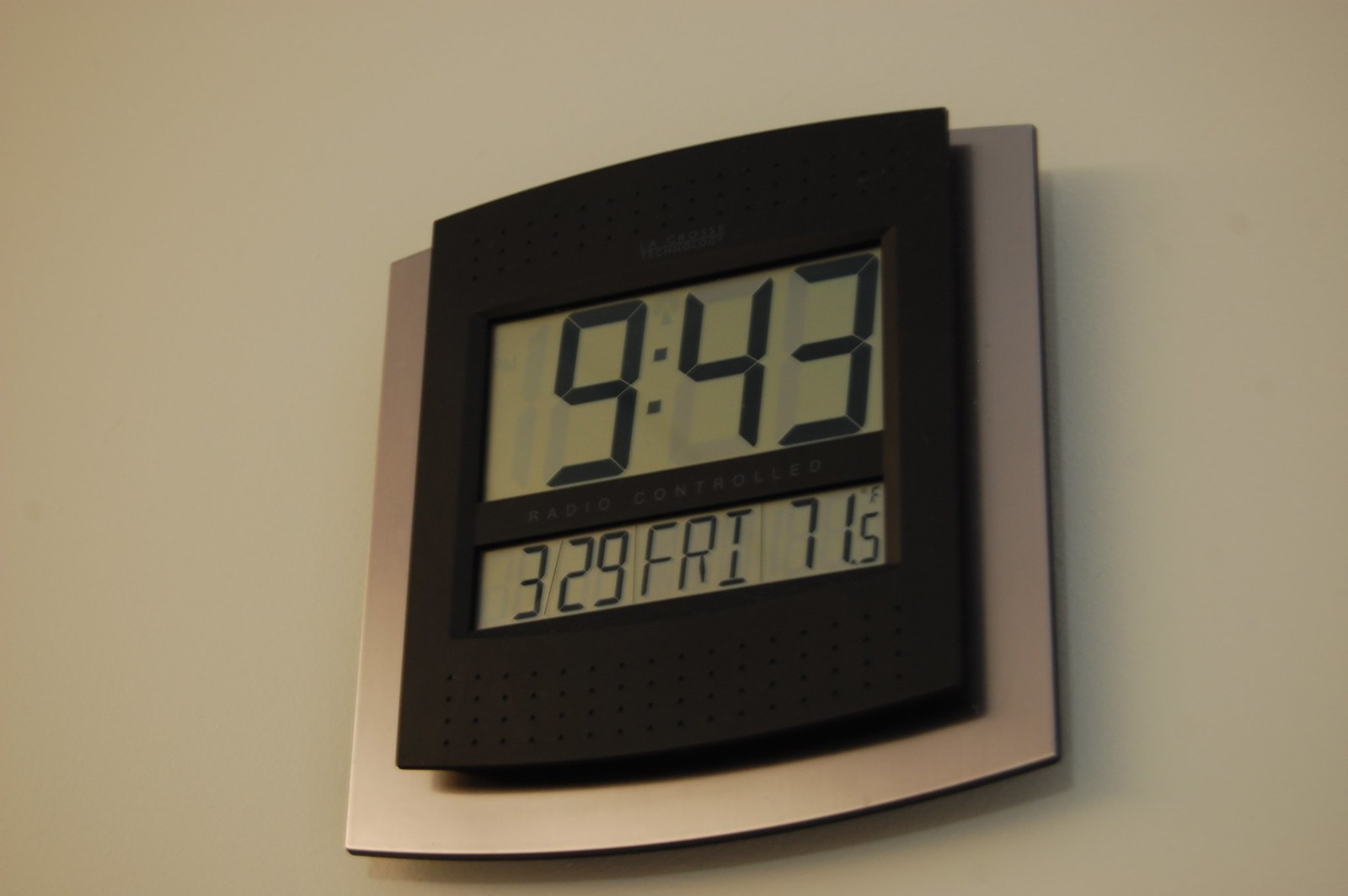A photograph captures a digital wall clock prominently displaying the current time as 9:43. The clock, which features a black front panel with a metallic casing, is reminiscent of those often seen in schools. Below the time, the clock's display indicates "Radio Controlled" in white text. Further down, another screen shows additional information: the date, March 29th (Friday), and the ambient temperature, 71.5 degrees Fahrenheit. The clock casts a subtle shadow on the wall behind it, which is painted in a typical whitish-gray hue. The image focuses solely on the clock, with no other discernible background elements, emphasizing its functional and straightforward design.